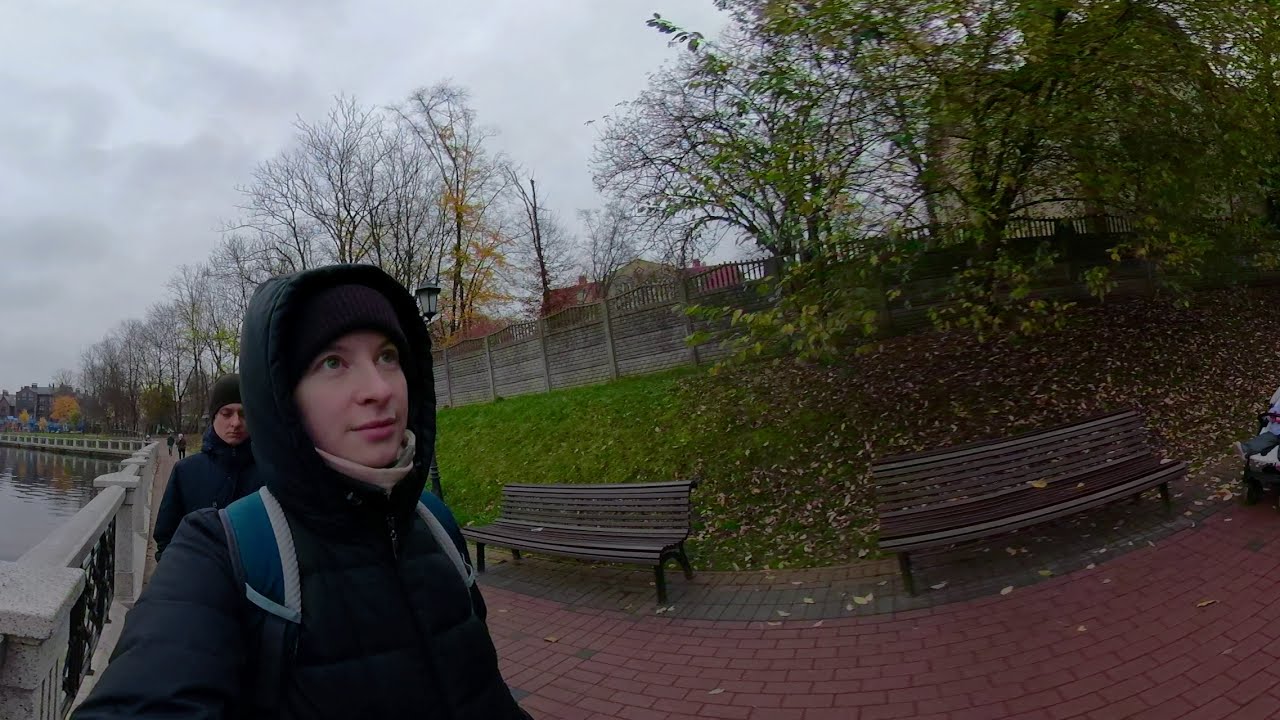In the chilly autumn weather, two women, warmly dressed in hats and jackets, stroll along a red brick walkway. The photograph, with its fisheye effect, distorts the immediate foreground where two curved benches sit on the terracotta surface. Surrounding the scene, a gray overcast sky looms, and the trees, half-naked with leaves scattered on the ground, hint at the seasonal change. A tall brick-and-wrought-iron fence lines the background, barely revealing houses and more trees beyond. To the left of the brick path, a concrete gate permits a view of a body of water below. One woman, wearing a popper jacket with a hood and a knitted toboggan, appears to carry a teal-strapped backpack. Her companion, similarly bundled up, walks just behind her.